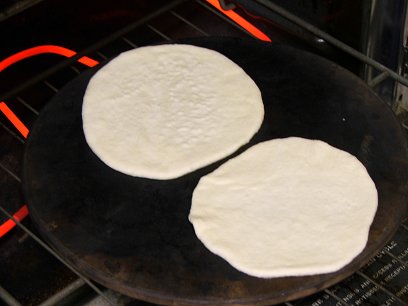The image depicts two uncooked tortillas placed on a round, weathered baking sheet with some brown and possibly rusted areas. The baking sheet rests on a wire rack inside an oven with bright orange heating elements visible in the background, indicating that the oven is on and quite hot. The tortillas appear freshly placed in the oven, as they have not yet started to brown and remain a pale beige color with visible dough spots. The left tortilla is beginning to show gentle bubbling on its surface. The round baking sheet under the tortillas seems slightly bent, curving upwards from the vantage point. The wire rack supporting the baking sheet is a dark grey or black color.